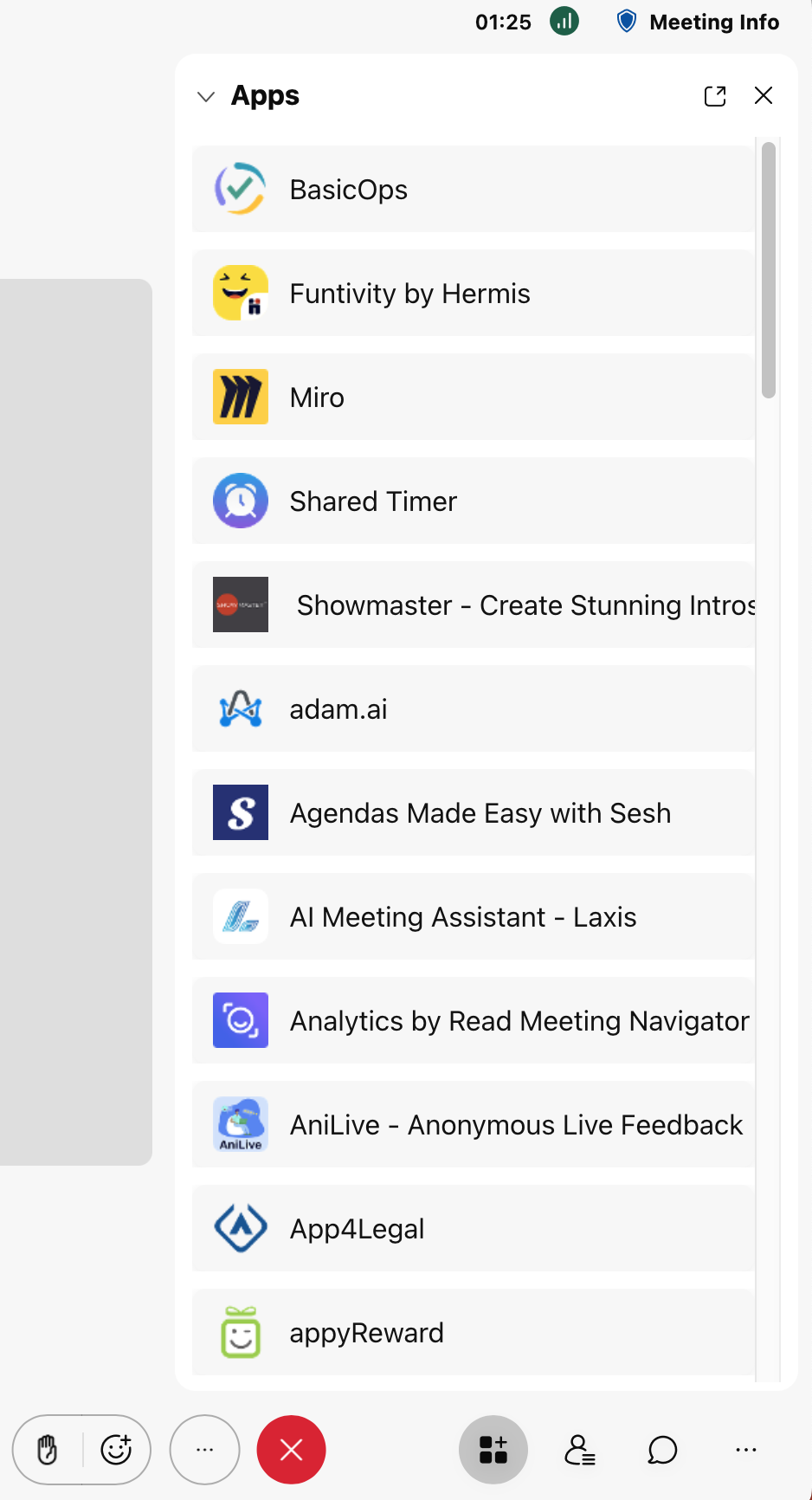In this screenshot, captured against a light gray background, we observe a user interface. At the top right corner, a light gray header displays the time "1:25" in black text and a "Meeting Info" label. Below this header is an opened pull-down menu in bold text titled "Apps." The menu items are listed in a structured format from top to bottom. 

1. **Basic Ops**
2. **Fun-tivity by Hermes**, accompanied by a yellow square icon with a smiley face.
3. **Miro**
4. **Shared Timer**, marked with an icon of a white alarm clock in a blue circle.
5. **Show Master, Create Stunning**
6. **Adam.AI**
7. **Agendas Made Easy with Sesh**
8. **AI Meeting Assistant Laxus**
9. **Analytics by Reed**
10. **Meeting Navigator**

Each item in the list appears with its respective icon and name, providing a clear and organized view of the available applications within this interface.